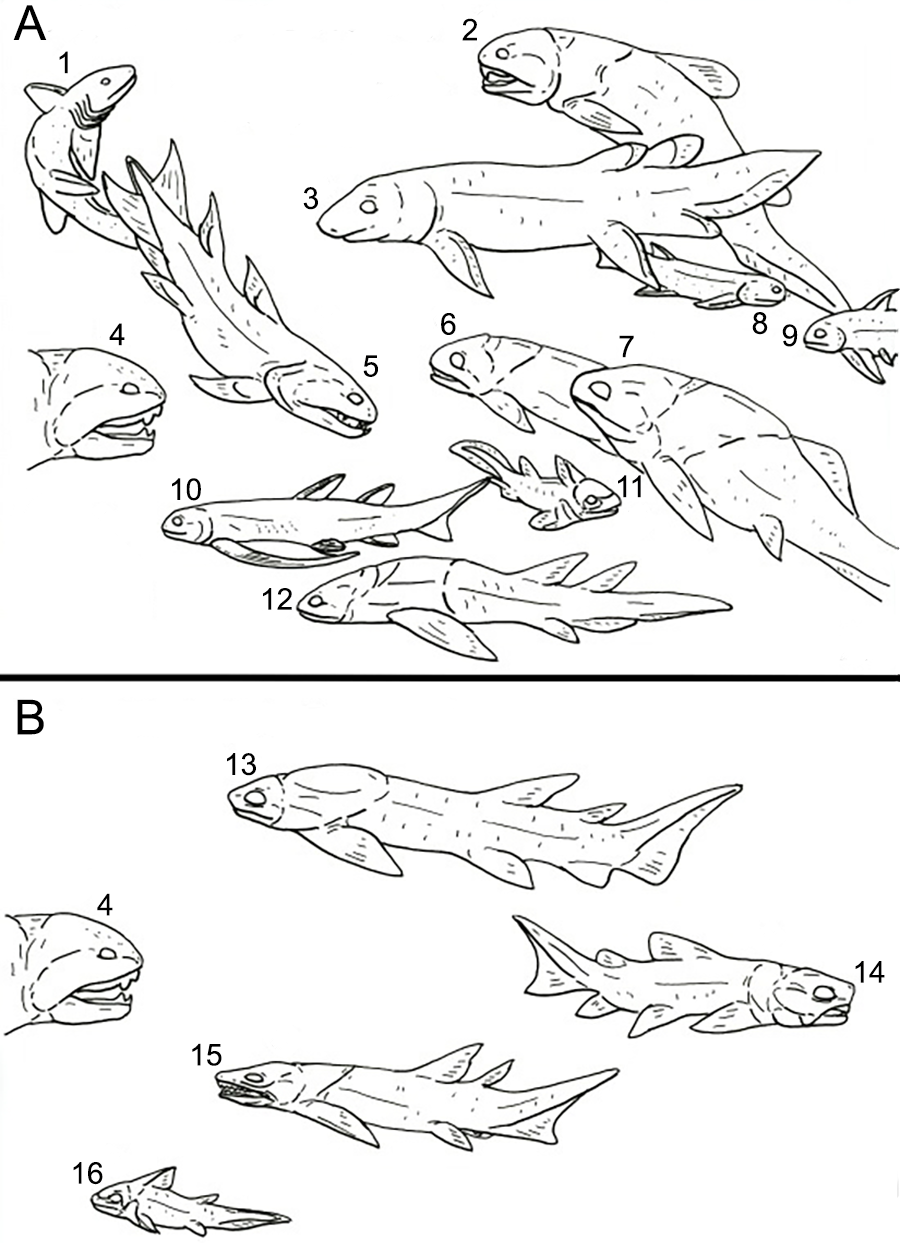The image is a detailed black and white drawing that appears to be from a textbook. It features two sets of fish illustrations on a white background, separated by a black horizontal line. 

In the top half, labeled "A," there are 12 fish drawings, each numbered from 1 to 12. These fish are drawn in black ink or pencil, and while they all look similar with simple, almost identical features, their positions vary.

Below the separating line, in section "B," there are 5 additional fish drawings, also in black ink or pencil. These fish are similar in appearance to those in section "A" but may have subtle differences such as the number of dorsal fins. Each fish in both sections is depicted in a straightforward, detailed style, suggesting an educational or scientific context.